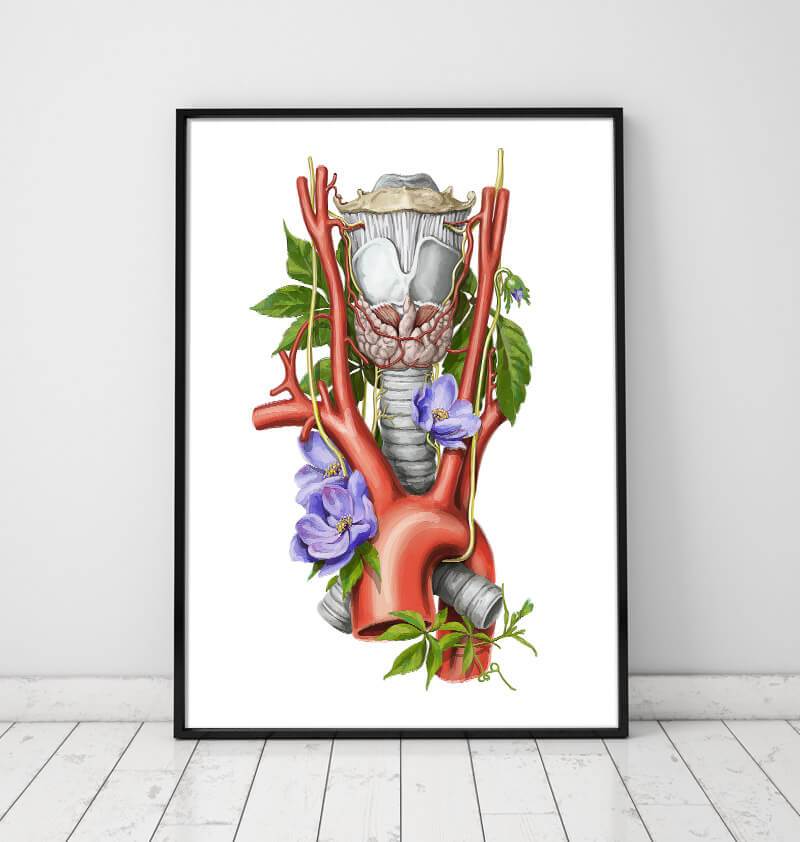The image showcases a detailed, computer-generated drawing inside a black picture frame with a white background. The drawing features a surreal blend of human anatomy, including arteries, a portion of a brain, tendons, skeletal sections, and internal body parts like intestines. These elements are intertwined with an organic array of green vines, leaves, and flowers. Specifically, purple and blue flowers are situated in various parts of the illustration—at the top and left, near the aorta and windpipe, and close to the jaw and eye areas made up of brain matter and hip bones. The overall scene is set against a white wall and a white wooden floor, with no other objects visible, highlighting the artwork's clarity and detail in the bright, natural light. There is no visible signature on the artwork.